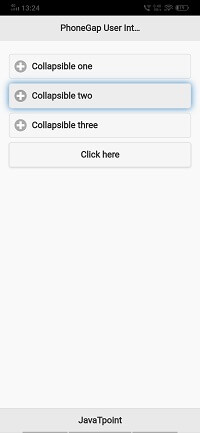The image depicts a screenshot from a phone displaying the "Phone Gap User Intel" interface. The top bar is very faint, making it difficult to discern the exact time, which appears to be in military format, either 1324 or resembling 21. Below the main header, "Phone Gap User Intel" is prominently displayed with black lettering on a dark gray background.

The interface presents three options labeled "Collapsible 1," "Collapsible 2," and "Collapsible 3," each accompanied by a plus symbol, indicating expandable sections. The user has seemingly highlighted "Collapsible 2," causing it to emit a blue glow around the selection, though it has not been expanded or clicked yet.

At the bottom of the screen, "Java T-Point" is displayed in dark gray text set against a lighter gray backdrop, making the text subtly noticeable. Overall, the interface is minimalistic and the color scheme relies heavily on various shades of gray and black, with minimal use of other colors, contributing to its understated appearance.